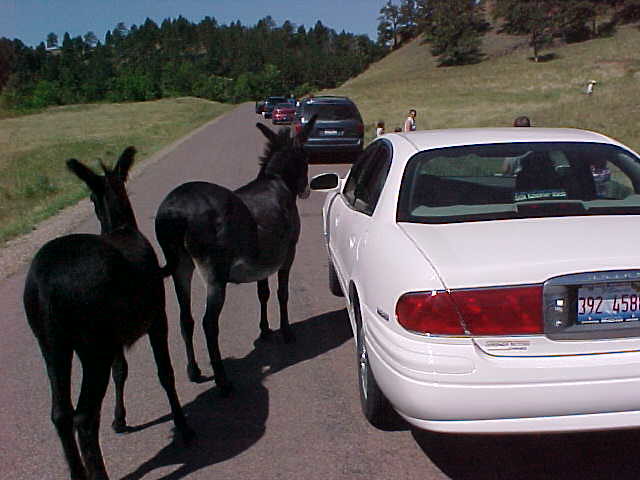The image shows a scene featuring two donkeys standing on a single-lane road, appearing to stop traffic. The donkeys, one in front of the other, have dark brown and black coloration on their legs. Positioned close to a white sedan, which is nearest to the camera, the donkeys are near the left edge of the image. To the right side of the frame, there's a hill with people walking up it. The background reveals a long, thin landscape with grass on the opposite side of the hill, suggesting this area might be a pull-off. Further along the road, visible through the trees forming a forested backdrop, you can see a line of cars, all stopped, possibly hinting at a traffic jam caused by the donkeys.